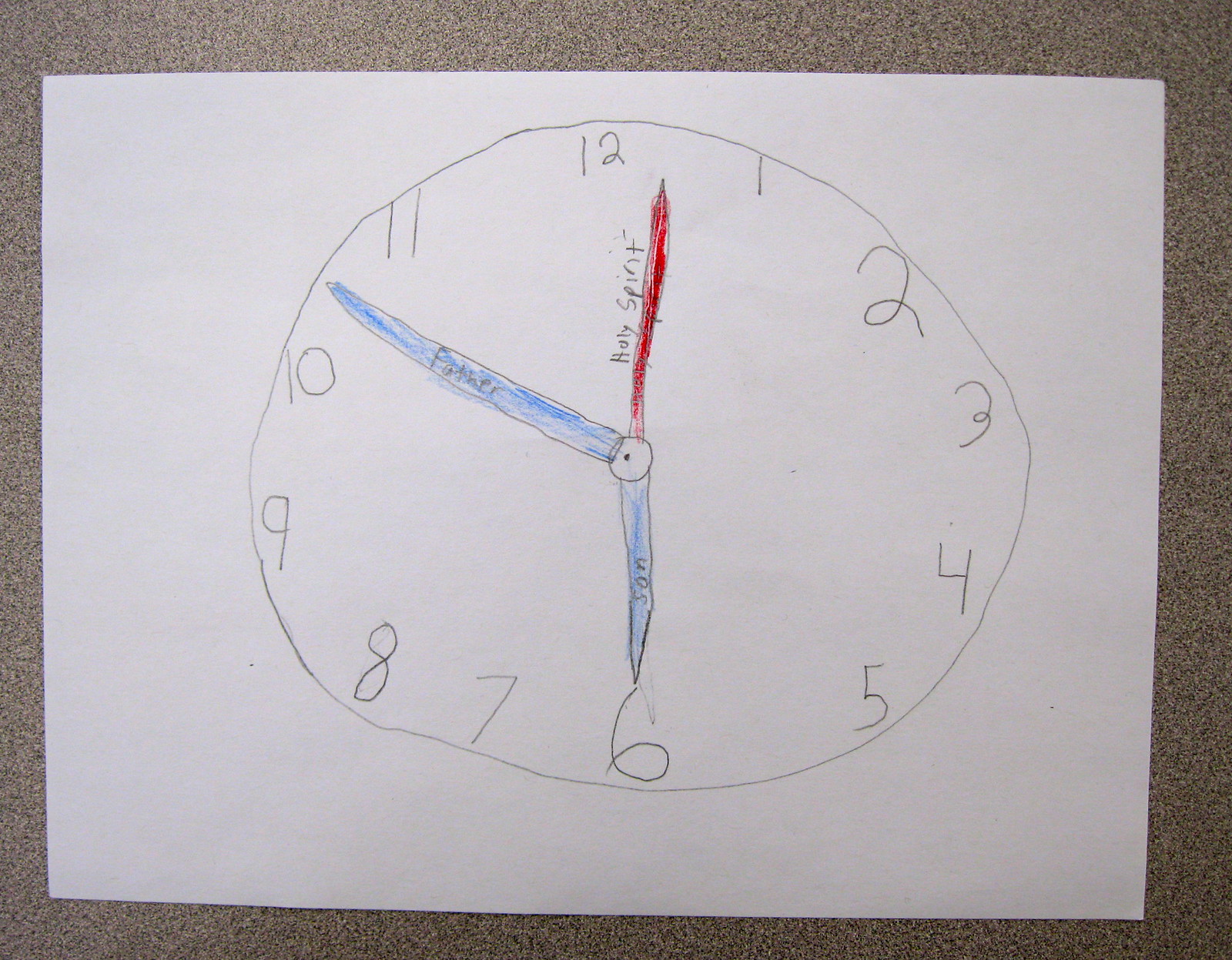On a blank white piece of paper, a round clock has been intricately sketched in pencil. The clock face features numbers 1 through 12 positioned at their respective hours. There are three hands on the dial: two blue and one red. The short blue hand, designated for the hours, is labeled "Sun." The long blue hand, indicating the minutes, is labeled "Father." The third hand, highlighted in red, represents the seconds and bears the label "Holy Spirit." Each labeled hand adds an element of symbolism to this thoughtfully detailed drawing.